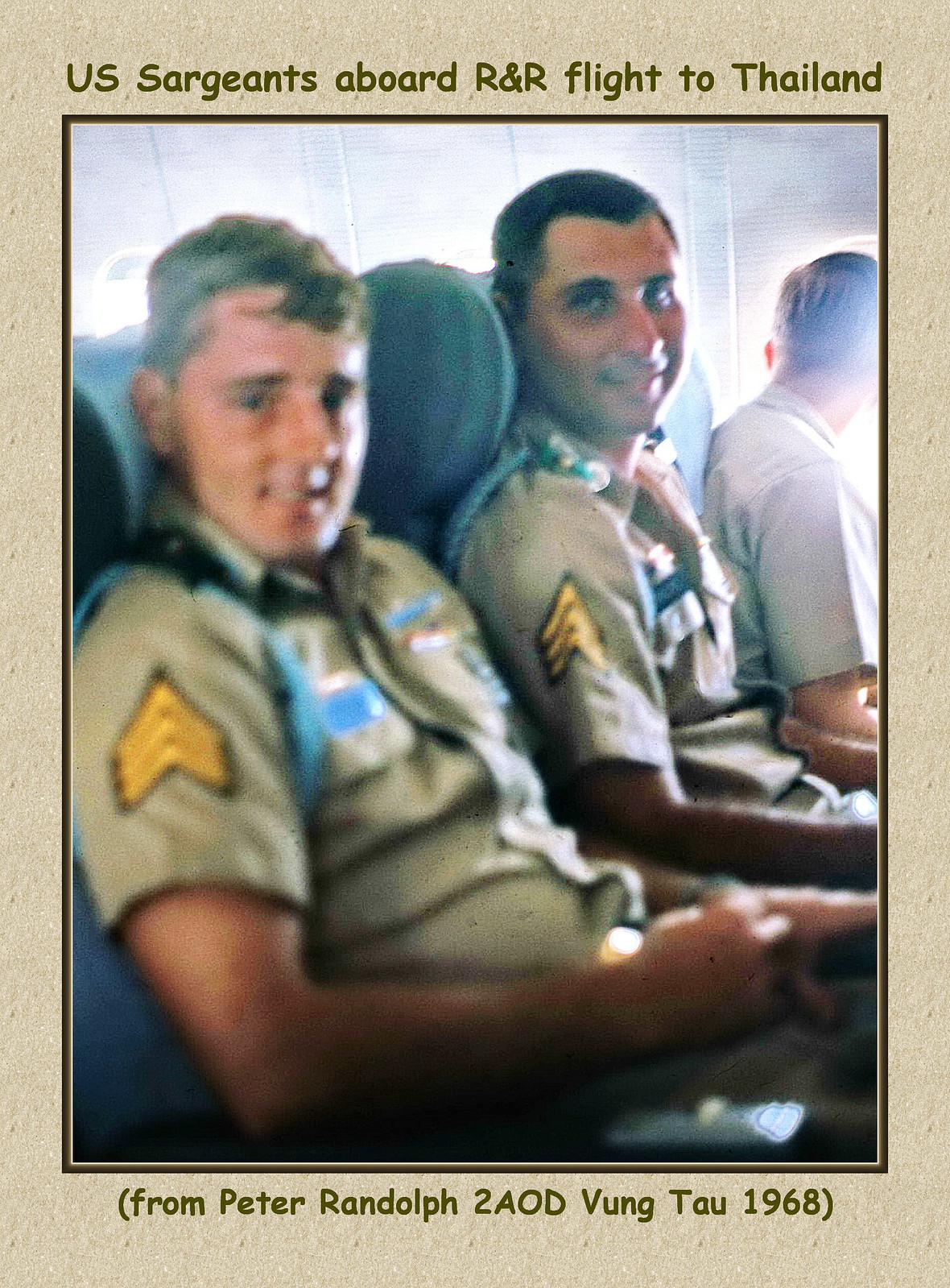This vertically aligned, rectangular photograph features a nostalgic and slightly blurry depiction of U.S. sergeants aboard an R&R flight to Thailand in 1968. The image is surrounded by a tan or brown border, with olive green text at the top reading, "U.S. Sergeants aboard R&R flight to Thailand." The bottom border bears the inscription, "(from Peter Randolph to AOD Vung Tau 1968)." Dominating the center, the photograph captures three men seated on an airplane with gray or blue seats. The two men in the foreground, likely in their late 20s or early 30s, both have short brown hair and are smiling at the camera. They are dressed in brown or khaki military uniforms, each adorned with a distinctive yellow inverted V-patch on their sleeves. Their hands rest casually in their laps. The man in the background, positioned on the far right, gazes out of the airplane window, his face partially obscured. The lively details and the content expressions of the men evoke a sense of camaraderie and historical significance amidst their journey.